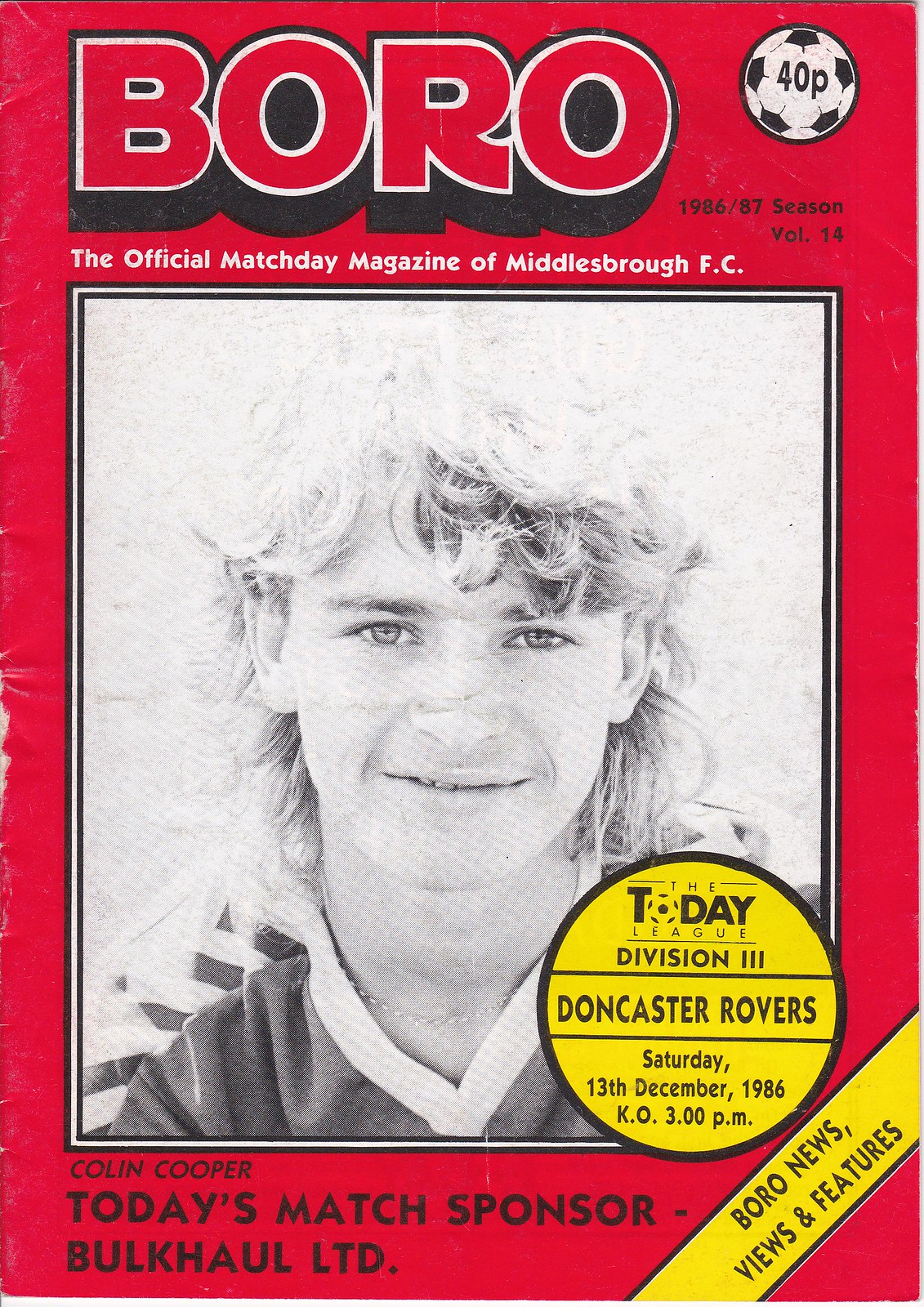The cover of the magazine features a solid red background with prominent text and imagery. At the very top, in red text with a thin white border and a thicker black border, it reads "Boro." To the right, a soccer ball contains the black text "40P." Below the soccer ball, in black text, it states "1986-87 season, Volume 14." A line of white text reads "The official match day magazine of Middlesbrough FC."

A large, black-and-white photograph of a young man, likely a soccer player, occupies the center of the cover. He has long, blonde hair that falls to the bottom of his neck and is smiling. He is wearing a V-neck style soccer jersey. On top of the photograph, there's a circle sticker with black text that reads "The Today League Division III, Doncaster Rovers, Saturday, December 13, 1986, K-O 3 p.m."

Below the photograph, text identifies the player as "Colin Cooper." Further down, it announces "Today's match sponsor: Bulk Hall LTD." The bottom-right corner features an angled yellow banner with the text "Boro News, Views and Features."